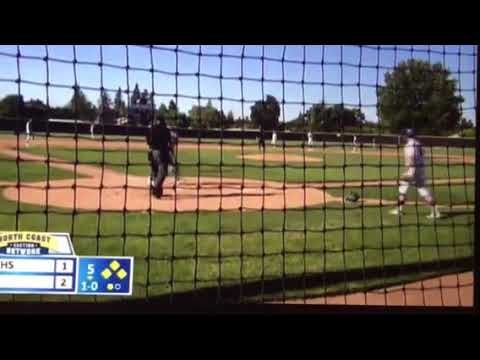This photograph captures a lively baseball game viewed through a protective black net positioned just in front of the camera, likely from a vantage point behind home plate. The game is set on a vibrant green field, framed by lush trees and a clear, sunny sky without any clouds. Positioned within the field of view are the umpire, garbed in a black shirt and gray pants, and a catcher, ready in his position. A batter, dressed in a light-colored uniform, stands poised to approach home plate. The baseball diamond's sandy base paths contrast with the surrounding verdant grass. In the lower left corner of the image, a blurry scoreboard is visible, possibly displaying the score 1 to 2. The scoreboard appears superimposed, suggesting it might have been added digitally or is a distant part of the scene, partially displaying the name "South Coast" before being obscured.